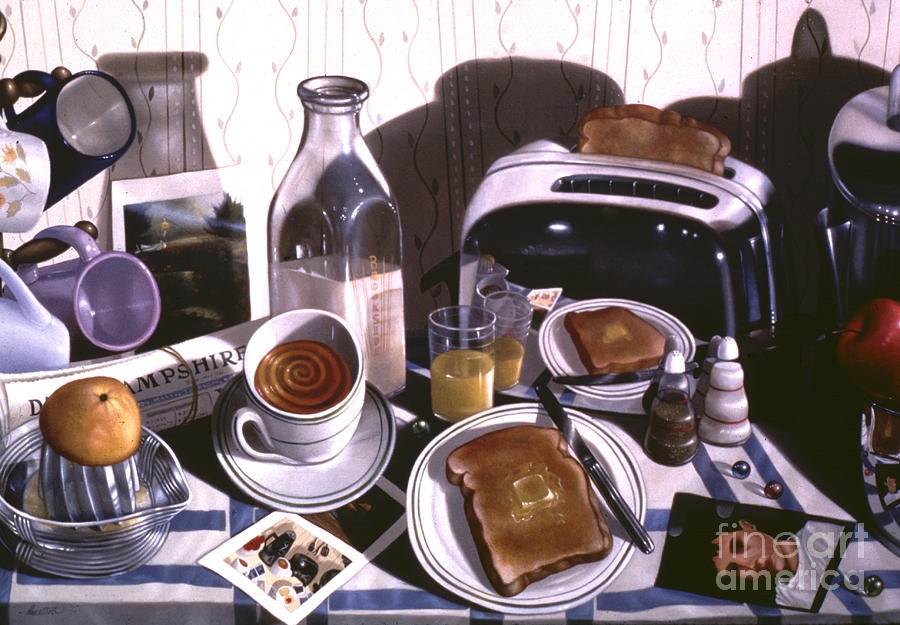The image is a detailed painting of a bustling domestic breakfast scene, reminiscent of an older style of artwork. The table is adorned with a white tablecloth featuring blue stripes and is laden with a variety of breakfast items. Central to the scene is a busy table setting, including a mug of coffee with a swirl design, a glass of orange juice, and a teacup and saucer filled with a brown liquid. There’s also a glass bottle of milk and a transparent jar with a cream-colored liquid. Toast features prominently, with buttered slices on a white plate and more pieces popping out of a shiny silver toaster. An assortment of breakfast essentials, such as an apple, an orange on a plastic juicer, and a lemon squeezer, add to the sense of an inviting morning meal.

The left side of the table shows a mug tree holding white and blue mugs, as well as a white mug with a floral design. A rolled-up newspaper, wrapped with a rubber band, rests nearby. The right-hand side contains a bread knife and a white plate with a slice of bread. There's also a picture of a man in white, a transparent container with white and brown powdery substances, perhaps for sugar and coffee, completing the scene. The background features patterned wallpaper and an image that evokes a country setting, adding a homely touch to this professionally crafted piece of art. The painting is signed "Fine Art America" in the bottom right corner, suggesting it may be part of their collection.